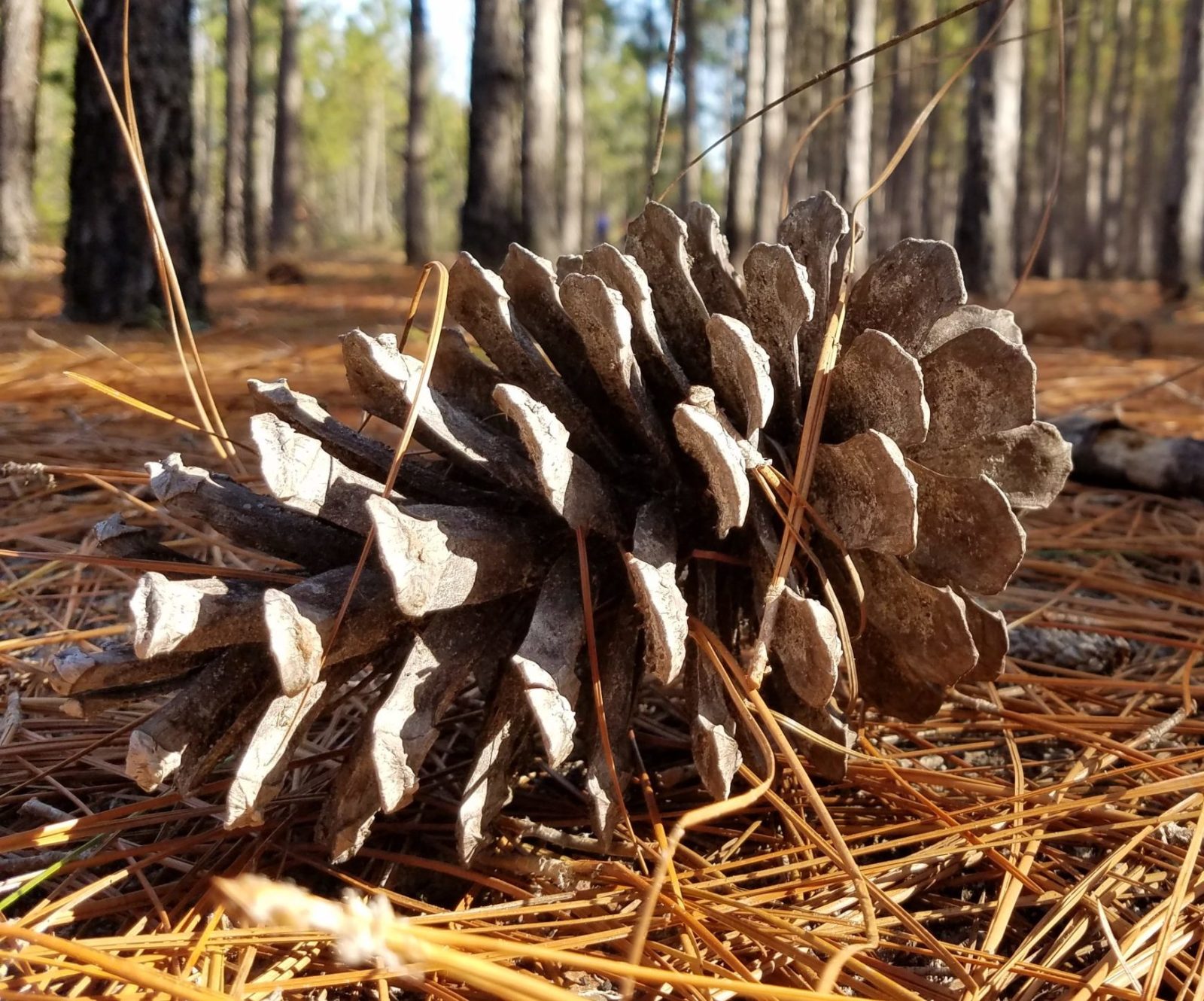This close-up, photorealistic image captures a large, rotted pine cone that dominates the central portion of the frame, occupying more than 50% of it. The pine cone, which displays grayish and brownish hues, lies amidst a bed of dead, yellow, and brown pine needles and straw on the forest floor. In the background, an array of tall trees with green leaves is visible, though blurred, giving depth to the scene. Scattered pieces of dead wood add to the forest's autumnal tapestry. The natural daylight filtering in highlights the textures and casts shadows, emphasizing the intricate details of the pine cone and the surrounding debris.